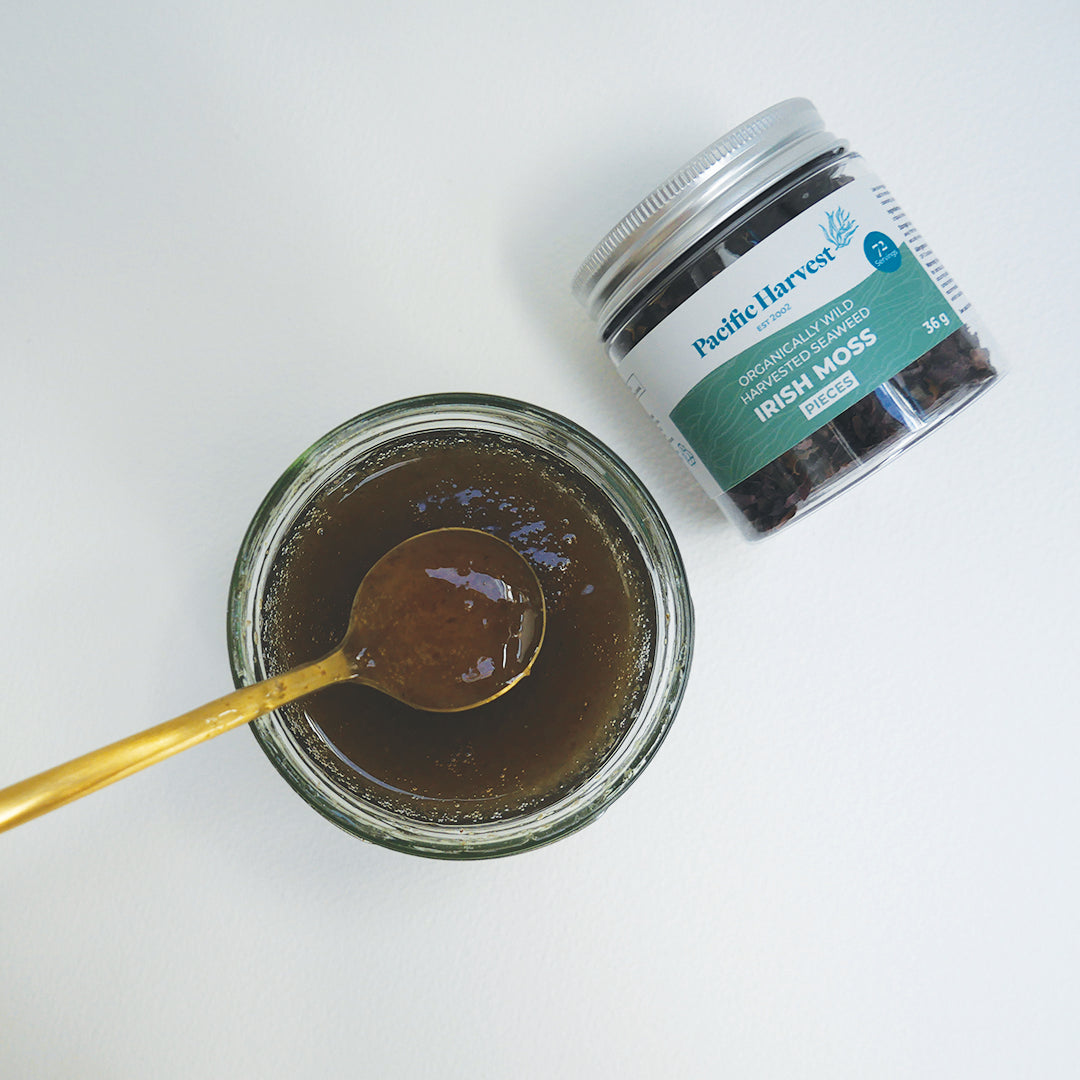The image showcases a health food product with a clean, white background, providing a clear bird's eye view. At the center, there's a glass jar containing a thick, brownish substance with a gold spoon inserted into it, overflowing with the same jelly-like material, giving it a honey-like appearance. To the right of this jar, positioned diagonally in the upper right corner, lies another glass jar tipped on its side, allowing for a clear view of its label. The label reads "Pacific Harvest, Organically Wild Harvested Seaweed Irish Moss Pieces," indicating it contains dried seaweed. Both jars are likely related, featuring the same seaweed product in different forms – one dried and the other in a more gelatinous, liquid state. The label specifies it has 72 servings, suggesting that these products are designed for health and wellness purposes.